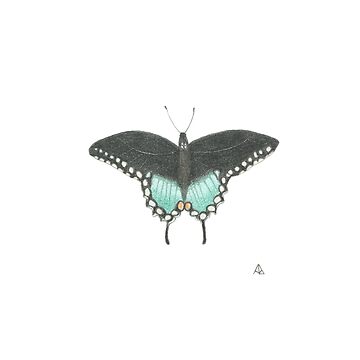This is an illustration of a butterfly on a plain white background. The butterfly is depicted with its wings outspread, appearing as a highly detailed pencil drawing. Its body is dark gray and long, with two black antennae extending from its head. The wings exhibit a striking color pattern: the upper portions are black, transitioning into a vivid turquoise at the bottom. Along the bottom edges of the wings, there are white circular shapes that stand out, except near the body where the last two circles turn orange. The entire illustration is symmetrical, highlighting the careful attention to detail in the wing patterns and body structure. The bottom of the wings also feature additional appendages reminiscent of a swallowtail, though the coloring and specific details suggest it is not an exact match to any known swallowtail species. There are no artist's signatures or marks.